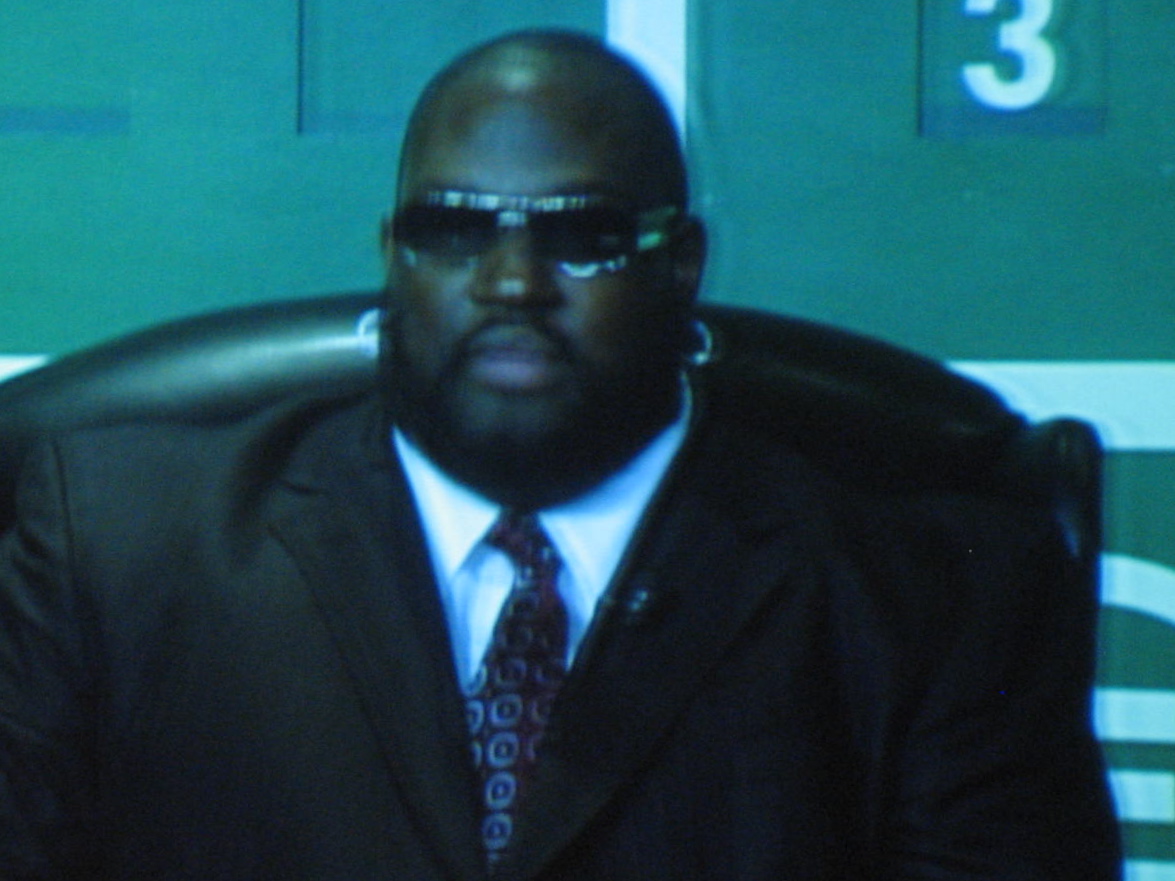In this close-up photograph, a bald African-American man with a neutral expression is sitting on a black leather chair. He is wearing dark sunglasses and has silver hoop earrings adorning both ears. His facial hair includes a mustache and a beard that frames his lips, though the area beneath his chin is ambiguous due to shadowing. He is dressed in a stylish black suit or tuxedo over a white collared shirt, accentuated by a red necktie featuring multiple Target logos in a dotted pattern. A small electronic device, possibly a microphone, is clipped onto his tuxedo jacket. The background showcases a vibrant green wall adorned with white stripes and banners, along with a prominently displayed white number “3” in the top right corner, indicating that the image might be a screenshot from a video owing to its slightly blurry and ghosting appearance.